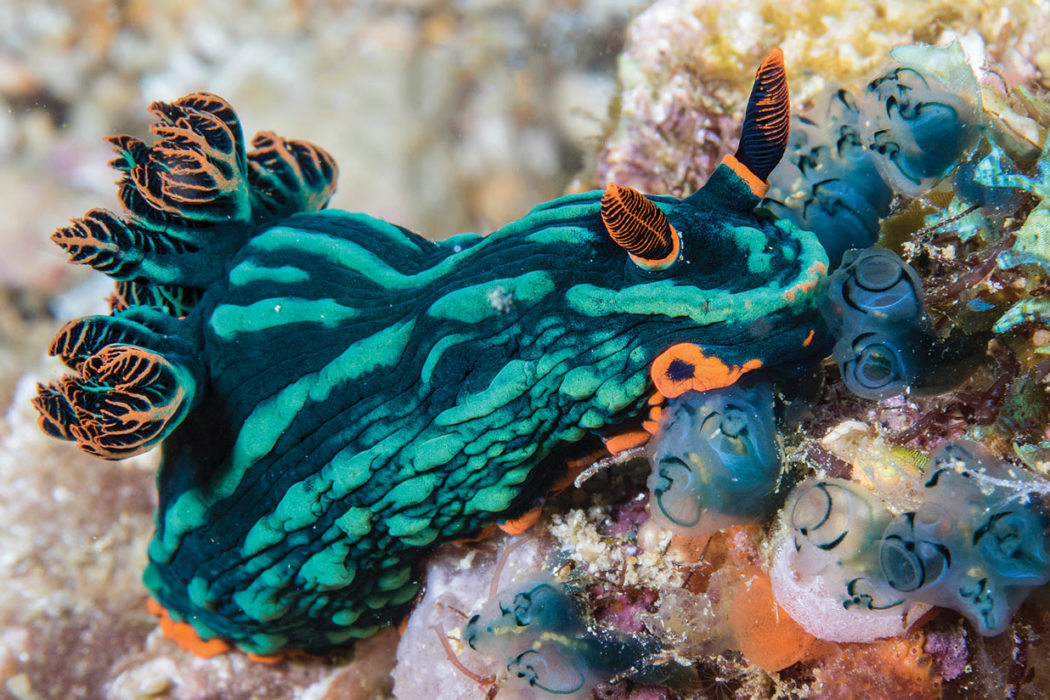The image captures a vibrant underwater scene featuring a nudibranch, a marine creature similar to a sea slug, photographed in what appears to be an aquarium or ocean setting. Predominantly, the nudibranch showcases two distinct shades of blue: a darker hue and a bright teal, with horizontal stripes marking its rough and warty body. The creature is accentuated with orange details along its lower side and two feathered, antenna-like extensions near its head that display a mix of black and orange. Towards the back of the nudibranch, there are additional appendages resembling branched coral, also adorned with orange and black. It is crawling over a light-colored, rocky seafloor, which is dotted with clear, ball-like, possibly sea anemones or similar growths in the lower right corner. The blurred background hints at more coral, keeping the focus sharply on the nudibranch.